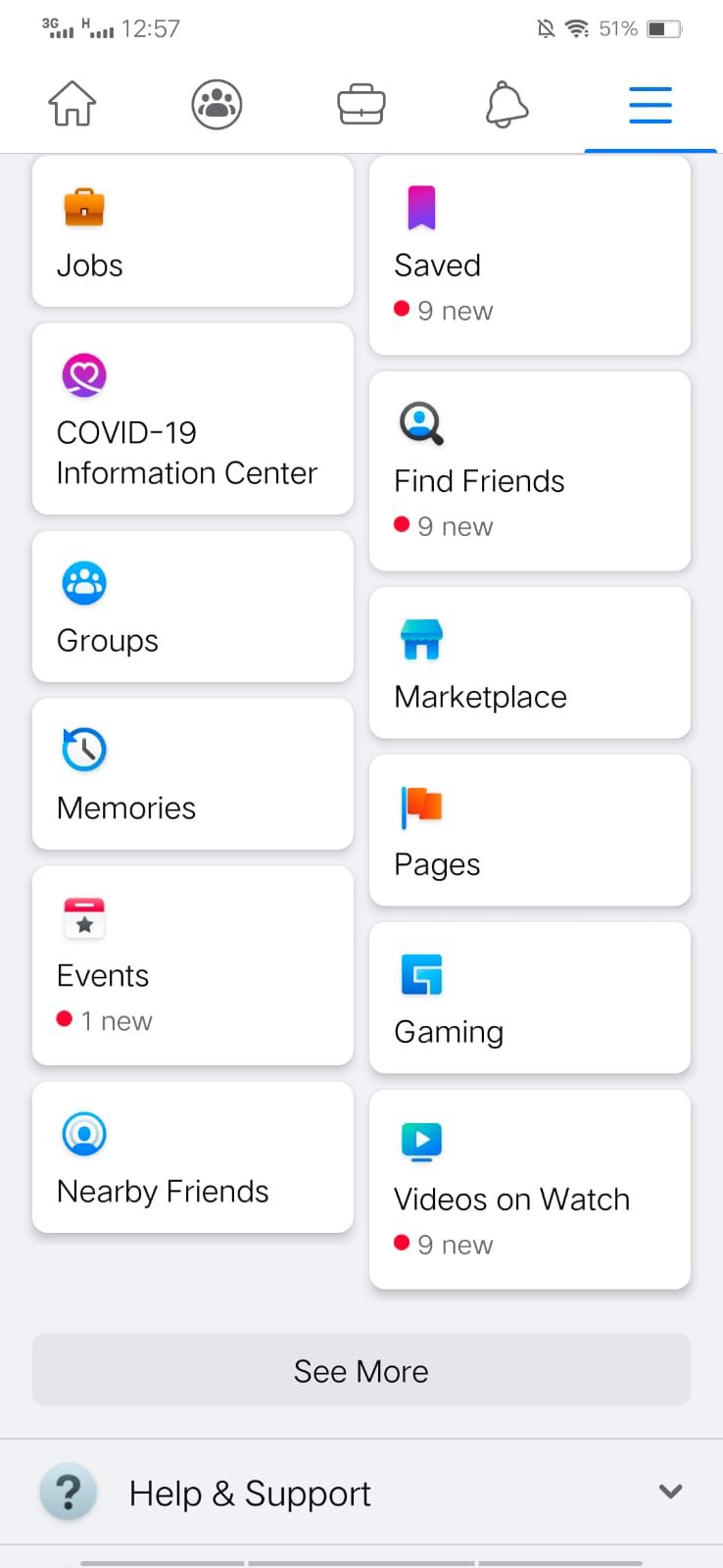This is a detailed vertical image screenshot taken from a smartphone. At the top of the screen, the status bar shows a 3G connection with signal strength bars, an 'H' indicator, the time displayed as 12:57, a muted alarm bell icon, a Wi-Fi symbol, and a battery icon indicating 51% charge.

Below the status bar, on the left side of the screen, several interface icons are present: a home button, a circle with a group of people, a bag or luggage icon, a bell icon, and a menu icon represented by three horizontal lines. These icons are highlighted in blue and have a blue underline beneath them.

The main part of the screen has a gray background with a series of rounded white rectangles, each containing an icon and a label. These labels include "Jobs," "COVID-19 Information Center," "Groups," "Memories," "Events," and "Nearby Friends." 

In a second column, additional options are listed: "Saved" (with a notification of nine new items), "Find Friends" (also with nine new items), "Marketplace," "Pages," "Gaming," and "Videos on Watch" (again with nine new notifications).

Below this section, a darker gray rectangular box contains the text "See More" in black. At the very bottom of the screen, a question mark icon is labeled "Help & Support" with a downward arrow indicating a clickable option for further information.